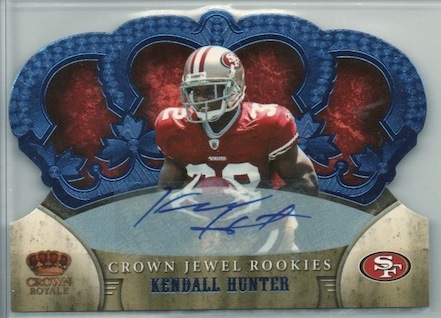The image depicts a unique piece of sports memorabilia featuring a football card designed in the shape of a crown. At the center stands a player for the San Francisco 49ers, identified as Kendall Hunter. He is depicted in a red jersey and full helmet, and his signature in blue ink is prominently displayed across the front. Behind him is an intricate crown design, colored in blue with red fabric visible through cutouts. Below the player, the card reads "Crown Jewel Rookies Kendall Hunter" in a gold section. To the left at the bottom, "Crown Royal" is inscribed along with a Victorian-style crown insignia, while the San Francisco 49ers logo in a red oval occupies the bottom right corner. The card is encased in a protective plastic case, suggesting it is well-preserved and likely unopened.